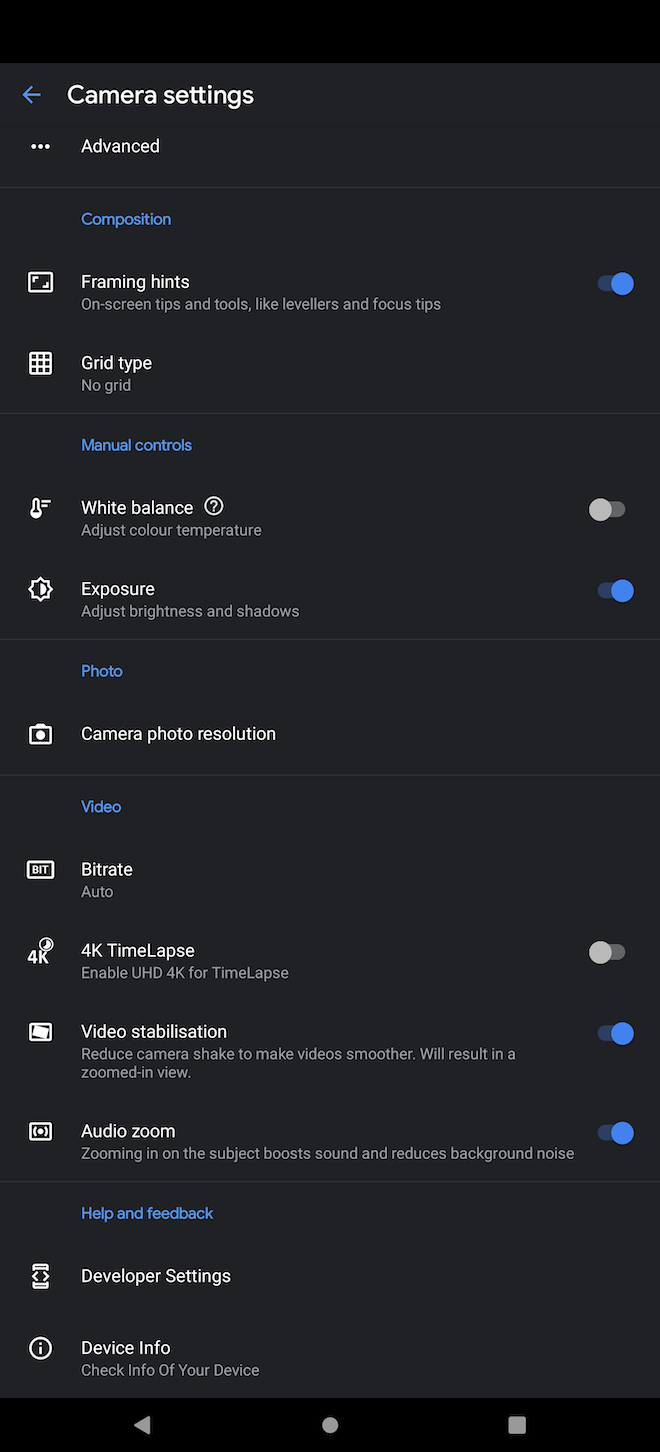The image portrays a detailed interface of camera settings. On the left side, an arrow labeled "Camera Settings" points towards an advanced composition section. This section is highlighted with dashed green lines and includes "Framing Hints," tips and tools such as levelers, and focus aids.

The interface shows various toggled options: 
- Grid Type: No Grid selected
- Smaller blue text at the bottom reads "Manual Controls"
- Larger text indicates "White Balance" with an option to adjust color temperature, which is not toggled.
- "Exposure" adjustment for brightness and shadows is toggled on.

Below, the "Photo" section displays options for camera photo resolution. In blue text next to this, "Video" settings can be selected. This includes:
- Bit Rate Audio settings, followed by an icon with the letters "BIT" inside a square.
- Options for 4K resolution:
   - "4K Time Lapse" (not toggled) with a description to enable 4K for time-lapse videos.
   - Video stabilization: reduce camera shake for smoother videos.
   - Zoom to Video, which is toggled on.
   - Audio zoom: zooming in on the subject boosts sound and reduces background noise, also toggled on.

At the bottom, it offers sections for "Help and Feedback," "Developer Settings," and "Device Info" for checking device information. Left and right navigational arrows are indicated with a circle at the center and a square on the right, respectively. The entire interface is set against a black bar background at the bottom.